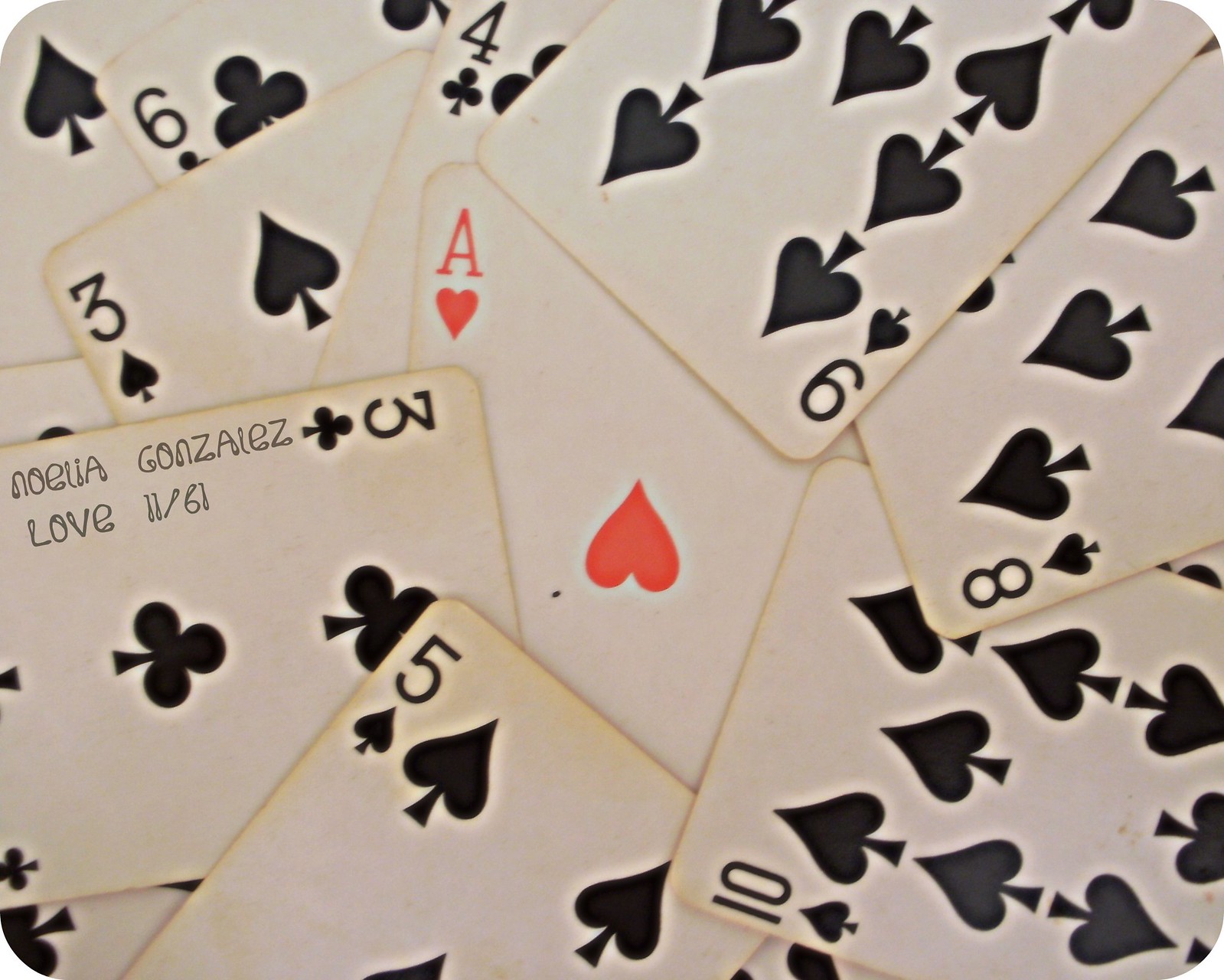Indoor, close-up, color photograph featuring a collection of approximately nine overlapping playing cards arranged face-up. Dominantly displaying the suit of spades, this photo's central focus is the Ace of Hearts. Starting at the upper left corner, part of the Six of Clubs is visible, oriented diagonally. Directly below it, the Three of Spades appears with its number positioned in the upper left corner, also angled slightly. Just left of the center, a partially obscured Four of Clubs peeks out. Directly to its right lies the Nine of Spades. The Eight of Spades enters the frame from the right edge, about halfway visible. From the lower right corner, the Ten of Spades is partially seen. Coming in from the lower left edge is the Five of Spades, while a Three of Clubs, featuring handwritten script "noeliagonzaiez," the word "love," and the number "1161," emerges prominently from the lower left. At the heart of this stacked and overlapping arrangement sits the unmistakable Ace of Hearts, serving as the central hallmark of this engaging card collection display.